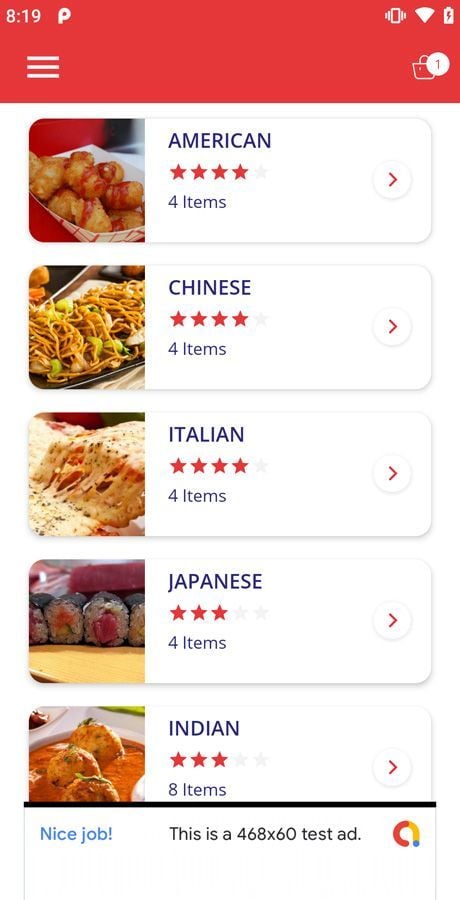On the screen of a phone, the user appears to be in the process of ordering food. The top of the screen features a red strip with the time displayed as 8:19 on the left side. To the right, a 'P' symbol indicates that the phone is on vibrate mode, and Wi-Fi is connected with the battery icon showing that the battery is charging. Below this status bar, on the right side, there are three horizontal lines stacked above each other (probably a menu icon) and a shopping bag icon with a number '1' in a circle, suggesting one item in the cart.

In the main part of the screen, there are five food category entries, each with a photograph on the left and details listed to the right. The categories include:

1. **American** - Rated at four stars, featuring four items, with an arrow to the right.
2. **Chinese** - Rated at four stars, featuring four items, with an arrow to the right.
3. **Italian** - Rated at four stars, featuring four items, with an arrow to the right.
4. **Japanese** - Rated at three stars, featuring four items, with an arrow to the right.
5. **Indian** - Rated at three stars, featuring eight items, with an arrow to the right.

Below these entries, a black horizontal line separates the list from a highlighted section that says "Nice job" in blue text. There’s also an ad displayed which includes a colorful logo resembling Google's red, yellow, and blue colors arranged in a circular pattern, though notably missing the green color. The ad text appears fragmented, mentioning something about "sixty test ad," but it is not clear in its entirety.

Overall, the user is browsing various cuisines including American, Chinese, Italian, Japanese, and Indian food options on a food ordering application, though specific location and additional context are not provided. The colors visible in this display include red, white, blue, brown, and green.